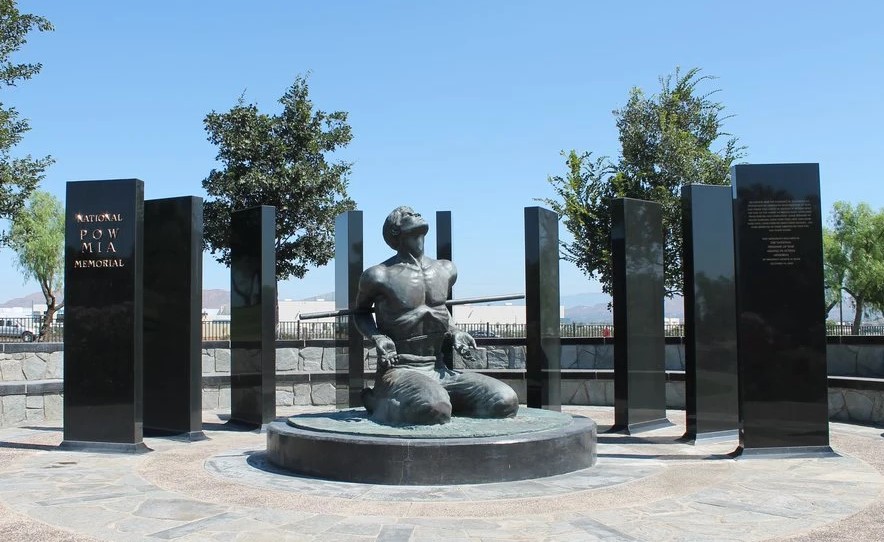This is a clear photograph of the National POW MIA Memorial taken on a bright, cloudless day with a brilliant blue sky. In the center of the image, set on a round, black marble platform, stands a hauntingly detailed sculpture of a famished man on his knees. The man, with his wrists by his sides and head tipped back staring up at the sky, has torn clothing revealing his chest and appears bound with ropes around his abdomen and wrists. This central statue is surrounded by nine sleek, black, obelisk-like pillars arranged in a semi-circular formation, each with inscriptions, including on the first pillar to the left which prominently displays "National POW MIA Memorial" in gold. The background of the photograph features a serene park setting with a few trees and distant, low-lying brown hills, while the ground beneath the monument is composed of large, light gray stone tiles, contributing to the solemn and reflective atmosphere of the memorial.